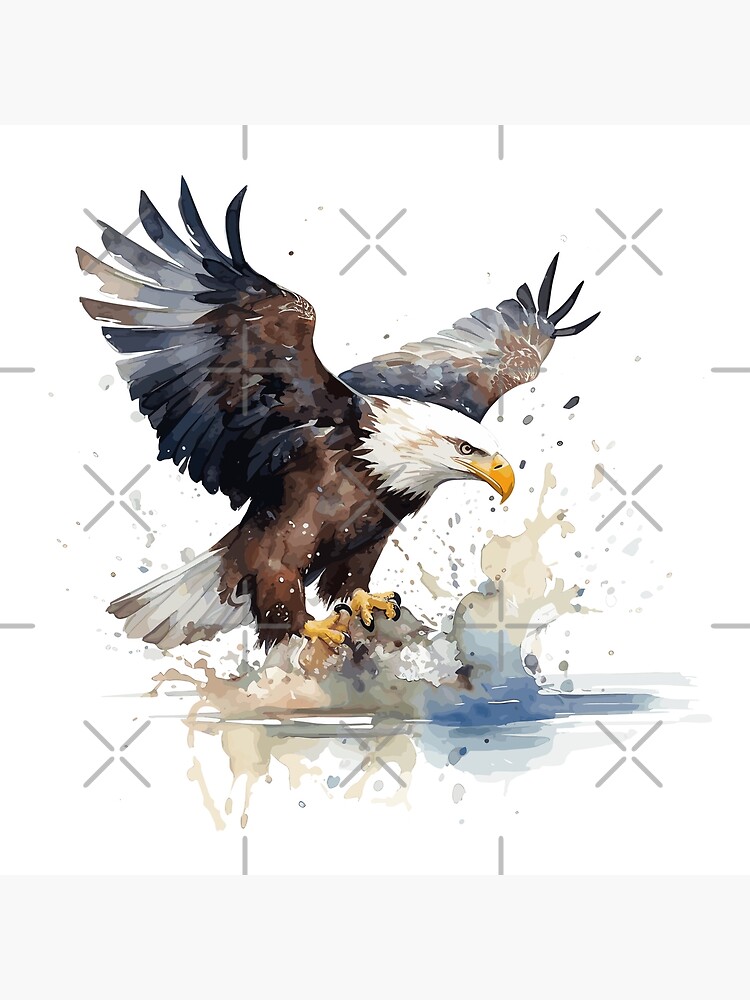This image displays a detailed digital illustration of a bald eagle swooping down towards the water, seemingly attempting to grab a fish or some other prey. The eagle’s body is predominantly brown, with certain portions of its wings highlighted in blue. Its head is distinctively white, complemented by a bright yellow beak and legs. As the eagle extends its claws towards the water, a violent splash is depicted, blending shades of blue and light brown. The perspective may appear slightly skewed, as the wing extending towards the viewer seems shorter than expected. The background of the scene remains entirely white, emphasizing the dramatic action in the foreground.